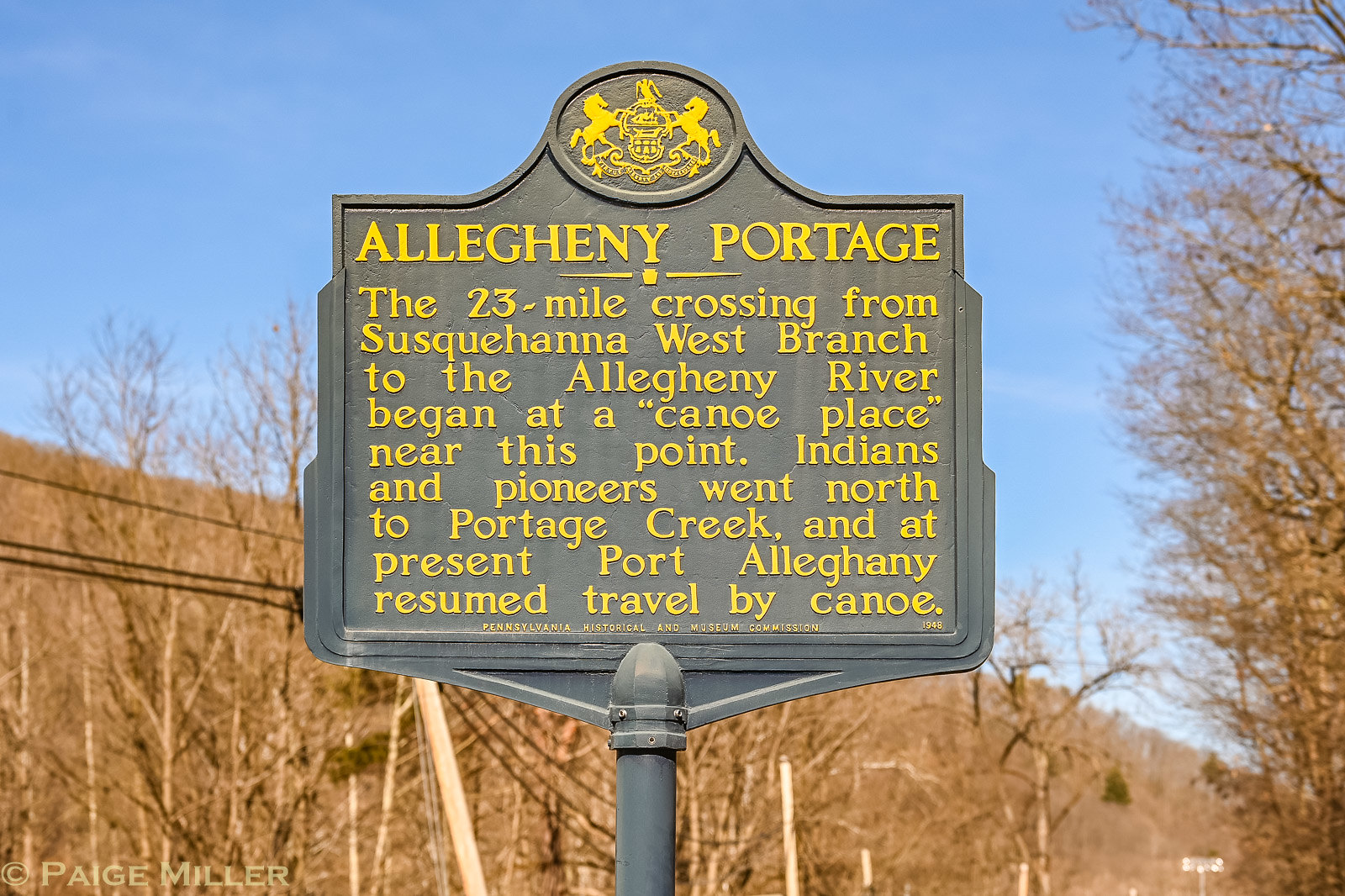The image is a landscape-oriented color photograph depicting a historical marker positioned at the center of the frame. The marker, which stands on a metal post, features a dark gray background with yellow typography and an intricate logo or coat of arms at the top. This emblem includes a gold horse on each side facing a shield, surrounded by elaborate decorations.

The sign reads: *"Allegheny Portage. A 23-mile crossing from Susquehanna West Branch to the Allegheny River began at a 'canoe place' near this point. Indians and pioneers went north to Portage Creek and at present Port Allegheny resumed travel by canoe."* In small print at the bottom, it is noted: *"Pennsylvania Historical and Museum Commission 1948."*

The scene is set in a sparse, wintry environment with numerous leafless trees and ragged vegetation, suggesting it might be late fall or winter. Most trees are bare except for one green pine tree in the background. The sky is clear and blue, providing a vivid contrast to the gray and yellow of the historical marker. The sign appears to be located near a hill, possibly by a roadside, and a wall is partially visible to the left, adding context to its historical significance and placement.